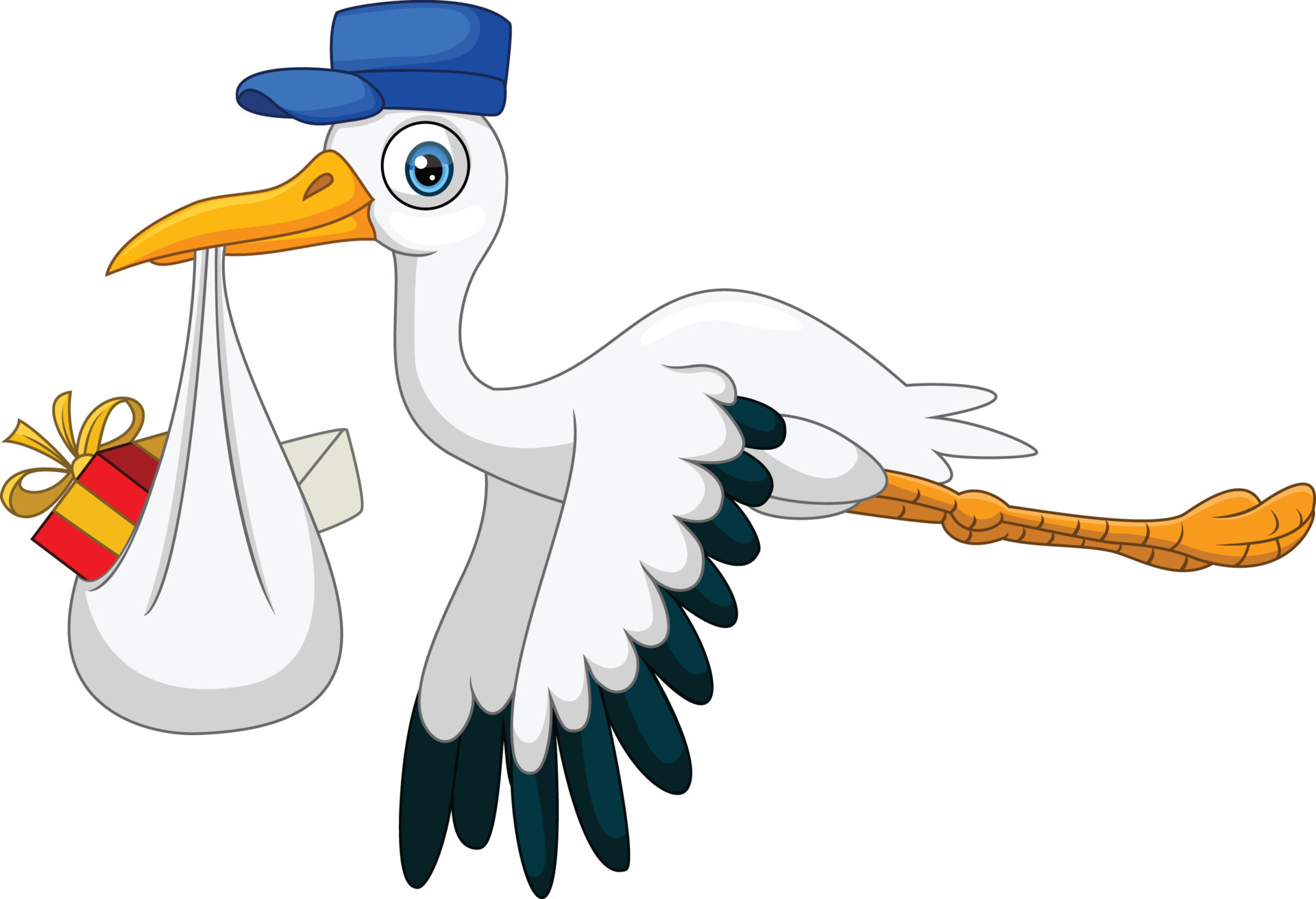The image depicts a detailed drawing of a stork flying towards the left against an all-white background. The bird is primarily white with bluish-green tips on its wings and orange legs extending backward with rounded knee joints. Its beak is long and yellow with darker yellow shading around the nostrils. The stork is wearing a blue cap with a black stripe, adding a whimsical touch to its appearance. Its eye is striking with layers: white surrounding a bright blue ring, a black pupil in the center, and a white dot indicating shine. The stork is holding a white cloth in its beak; this cloth has creases and contains a red and yellow gift with a golden ribbon. A hint of an envelope can be seen sticking out from the other side of the cloth.